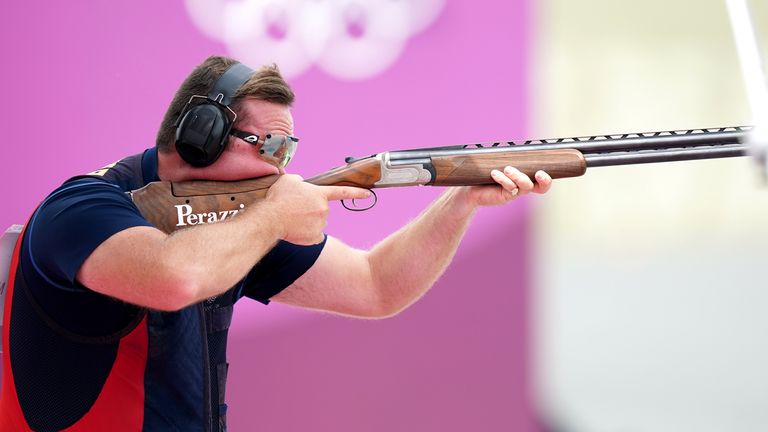In this photograph, a focused white man is seen aiming a Perazzi shotgun characterized by a long metallic barrel and a wooden handle. He is equipped with safety goggles and earmuffs for protection, emphasizing the seriousness of his task. His clothing consists of a short-sleeved blue shirt with red designs and a red vest, and he also sports a gold pinky ring. The man is positioned from left to right, with his finger near the trigger and his underhand supporting the barrel. The blurred pink background prominently features the Olympic rings, indicating that he is participating in an Olympic shooting contest.